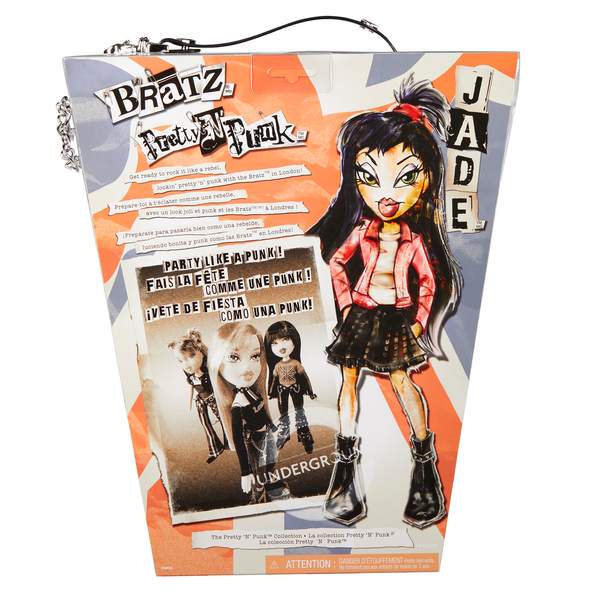The image showcases a vivid, punk-themed product packaging for a Bratz doll named Jade. The uniquely shaped packaging, resembling an upside-down trapezoid, features a silver chain link handle. The design prominently includes stylized, cut-and-paste text, giving it a rebellious, ransom letter aesthetic. "Bratz: Pretty in Punk" is emblazoned at the top, with "Jade" appearing in black and white cut-and-paste text on the top right.

On the right-hand side, there is an illustration of Jade, characterized by her dark hair with short bangs, a small ponytail held up by a red hair tie, expressive green eyes, and full red lips. She is dressed in a beige shirt, a red jacket, a short black pleated skirt, and chunky black boots adorned with silver studs around the ankles.

To the left of the doll's image, descriptive text details various features of the doll. Below this, a small poster showcases photorealistic images of the dolls with more cut-and-paste styled text that reads, "Party Like a Punk" in three languages: English, French ("Fais la fête comme un punk"), and Spanish ("Faites des fiestas comme un pooky").

The background features a vibrant red, white, and blue flag with a design reminiscent of the Union Jack, reinforcing the punk theme. Throughout the packaging, additional illegible text in the same cut-and-paste style adds to the chaotic, punk vibe of the product. The packaging’s palette includes orange, black, red, white, blue, gray, yellow, and whitish gray tones, further adding to the eye-catching nature of this Bratz doll's punk rock presentation.